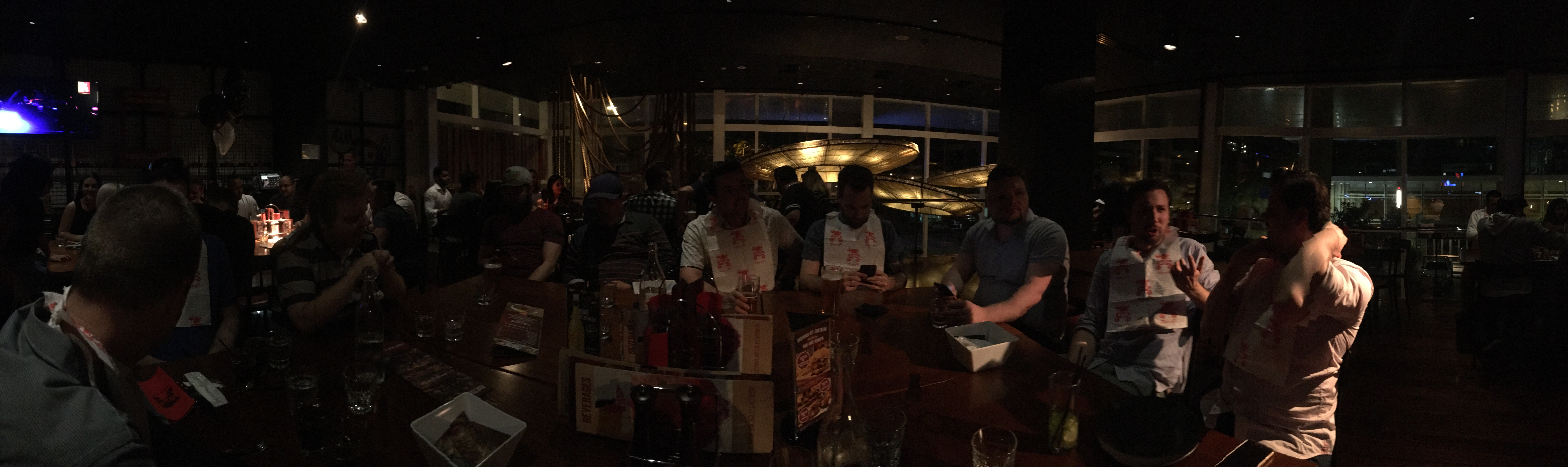In the dimly lit interior of what appears to be a bar or a restaurant, the image shows a scene teeming with subdued activity. On the left side of the image, a blue and white shade or reflection of light mildly illuminates the dark space, accentuating various glows and hues that give the place its moody ambiance. Against the right side of the room, five men are situated: a couple stand or partially sit at the bar, while more men occupy seats in the vicinity, creating a snug and social atmosphere. It appears there is a basin and an array of items cluttering the bar area. Deep in the background, windows hint at an additional seating area bathed in soft, ambient light possibly radiating from a distant source. This space is likely catering to customers indulging in drinks and conversations. There are containers and possibly beverages scattered around, alongside other paraphernalia that suggest a typical setting for a sports bar or a dining area in a casino. Moreover, a few individuals are adorned with bibs, hinting at the consumption of particularly messy cuisine. The collective gaze of some patrons appears directed toward the photographer, with others seemingly engrossed in watching television. Overall, the photograph encapsulates a lively yet intimate ambiance, where dim lights, reflective surfaces, and the muted buzz of activity blend seamlessly.